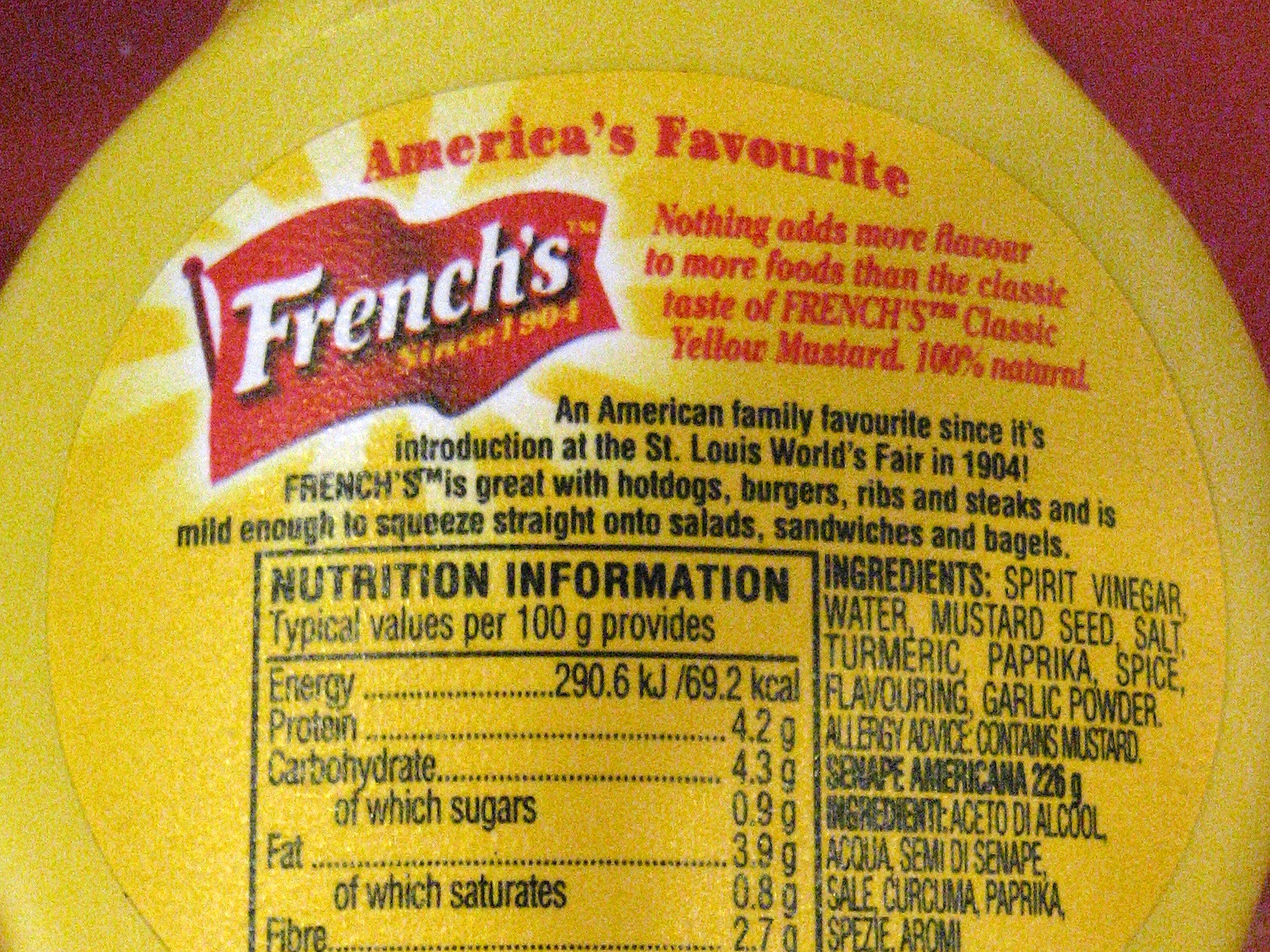A detailed, zoomed-in image captures the central portion of the label on the back of a French's mustard squeeze bottle. The familiar French's label is prominently displayed in the top-left corner, showcasing the brand's iconic red and white logo. Adjacent to the logo, bold text proclaims "America's Favorite," emphasizing the widespread popularity of this classic condiment. Below this, a brief description celebrates French's Classic Yellow Mustard as a beloved family favorite since its debut at the St. Louis World's Fair. The lower portion of the image features the Nutrition Facts box, outlining detailed nutritional information. To the right of this box, the ingredients list is visible, detailing the expected components of mustard. The photograph focuses solely on the central label, omitting the top and bottom parts of the bottle, thus emphasizing the informative and nostalgic elements of the product’s packaging.